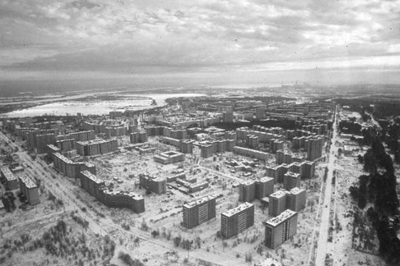This black and white aerial photograph, likely taken from a drone or aircraft, captures the haunting expanse of Chernobyl's desolate urban landscape. From an altitude of approximately a thousand feet, numerous tall, multi-story buildings stretch out into the distance, forming a stark cityscape beneath a sky dotted with puffy, speckled clouds and intermittent sunbeams. The ground, covered in a light-colored ash, adds to the eerie atmosphere, reminiscent of either snow or desert sand, obscuring the true nature of the terrain.

In the image, empty roadways and squares of the abandoned city are clearly visible, with a few distant vehicles, possibly trucks, whose movement status is indiscernible. The right side of the photograph shows denser clusters of trees, contrasting with the urban spread. In the distance to the left, a body of water—potentially a lake or river—glimmers faintly, hinting at what once might have been a harbor. The overall composition and desolation underscore the aftermath of the Chernobyl nuclear disaster, captured in stark, timeless monochrome.